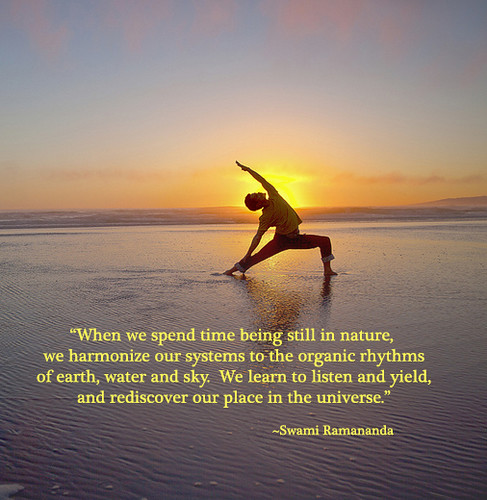The image captures a serene moment at either sunrise or sunset, with the sky painted in a harmonious blend of dusky hues, featuring shades of orange, yellow, light blue, and pinkish-purple. Dominating the scene, the glowing, golden sun is partially obscured by a slender, barefoot individual positioned in shallow, darker blue rippling water. This person, likely a woman, is gracefully performing a yoga pose. One arm is outstretched above her head, which tilts to the opposite side; her other arm reaches down to touch her ankle. She wears a light-colored, long-sleeve top that rides up slightly to reveal her midsection, paired with rolled-up jeans. The tranquil scene evokes a connection to nature, accentuated by the inspirational quote overlayed in yellow text at the bottom. It reads: "When we spend time being still in nature, we harmonize our systems to the organic rhythms of Earth, water, and sky. We learn to listen and yield and rediscover our place in the universe." – Swami Ramananda.